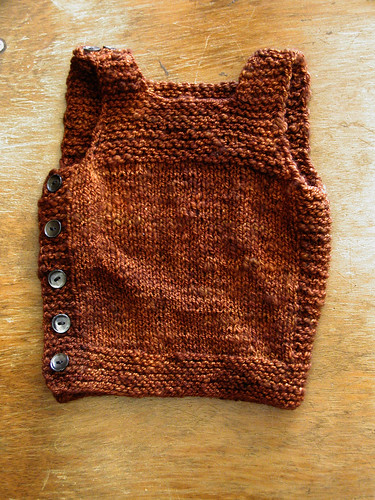The photograph captures a well-worn knitted vest, possibly a tank top, meticulously crafted from a bronze-brown or rust-colored yarn, and is lying on a beige wooden table. The vest displays a closely-knit pattern, with a distinctive change in stitching from the upper chest and shoulders down to the midsection. Notably, it features five silver buttons along its right side, which are evenly spaced. The seams around the armholes are visibly thicker, possibly reinforced or double-stitched. Despite some slight wrinkling from repeated use, the vest’s intricate craftsmanship is evident. The lighting casts a gentle reflection on the right side of the garment, highlighting its texture against the table’s subtle scratches and wear.